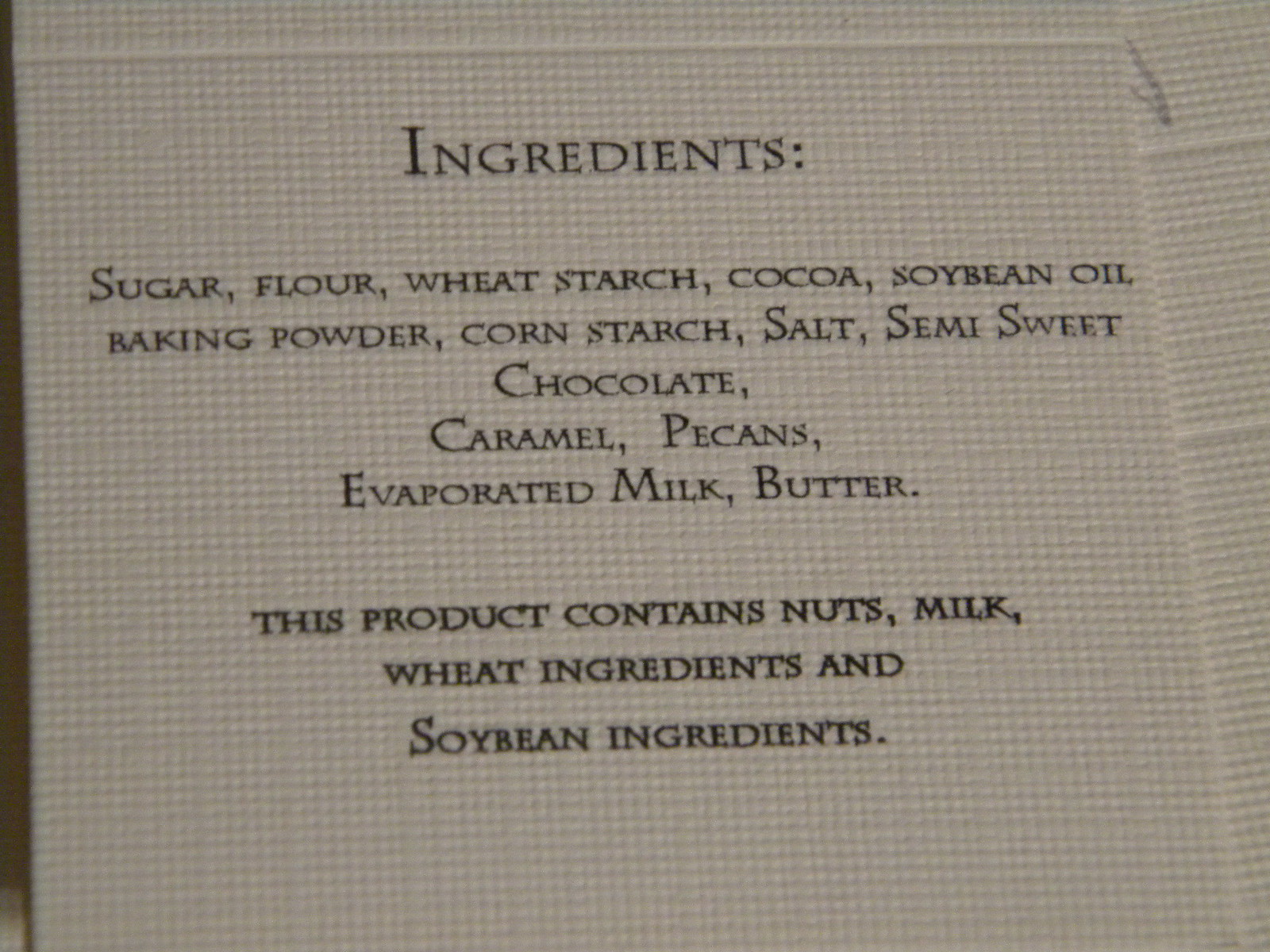This close-up photograph features a piece of white material with a bumpy texture, resembling cloth or possibly felt used for cross-stitching or as a backing for embroidery. The white background has a grid of small holes, reminiscent of braille or a textured paper. In bold black text, the material is printed with an ingredients list. At the top, it reads "INGREDIENTS:" followed by "Sugar, Flour, Wheat Starch, Cocoa, Soybean Oil, Baking Powder, Cornstarch, Salt, Semi-Sweet Chocolate, Caramel, Pecans, Evaporated Milk, Butter." Below this list, there is a notice in the same bold black text that states, "This product may contain Nuts, Milk, Wheat Ingredients, and Soybean Ingredients." The setting suggests a unique presentation style, possibly mimicking the format of product packaging but crafted on a piece of fabric.